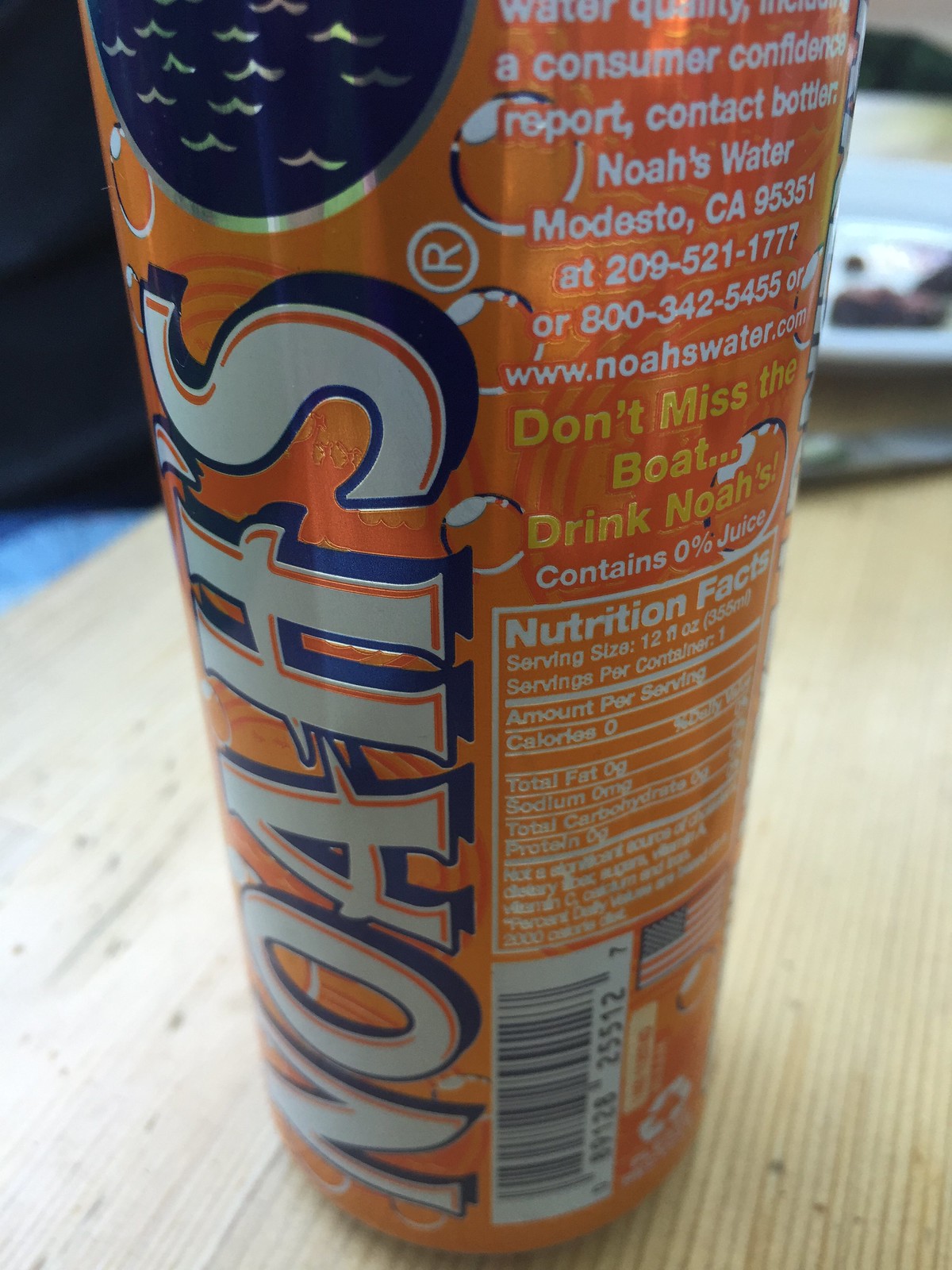This image showcases an aluminum can of water, distinctly marked as "Noah's." The can is slender and cylindrical, painted in a vibrant orange hue. Prominently featured is the Noah’s logo, which consists of blue and silver ocean waves adding a refreshing maritime touch. The can is partially rotated to reveal the barcode and some nutritional information, indicating that the beverage inside is water with zero calories and measures 12 fluid ounces.

Further details on the label confirm the water quality, including a consumer confidence report with contact information for Noah’s Water located in Modesto, California. Also visible are a phone number and a website for additional information. The can embraces an eco-friendly message with a slogan, "Don't miss the boat, drink Noah's," and displays both an American flag and a recycling logo, emphasizing patriotism and environmental awareness.